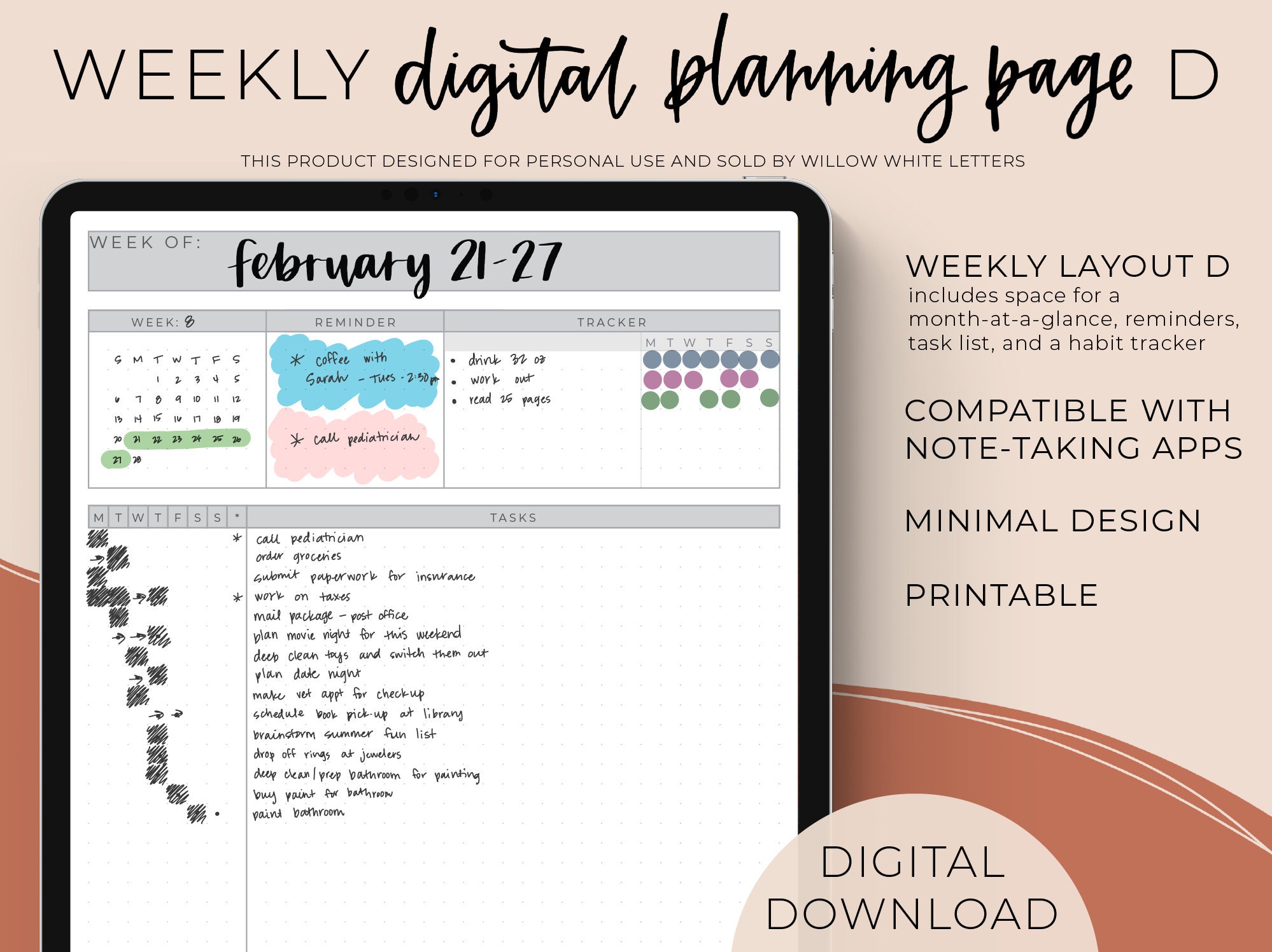This digital ad for a weekly planner features a sophisticated mock-up displayed on a device, likely an iPad, set against a light beige background that transitions into a darker brown graphic at the bottom. The showcased planner page, framed in black, highlights the week of February 21st to 27th. It includes essential sections such as a month-at-a-glance calendar with the week highlighted in green, reminders, a tracker, and tasks neatly arranged in a grid layout from Monday to Sunday.

At the top of the planner page is a gray bar marking the date range, followed by another horizontal gray bar segmented into columns. These columns include a month view, colorful blobs of text (illegible due to size), and different colored circles, indicating various planner features. Below these, a handwritten-style column lists tasks for each day.

The splash screen header prominently displays "WEEKLY" in bold sans serif text. Adjacent to this is the phrase "DIGITAL PLANNING PAGE" in handwritten text alongside a large capital "D" in a matching sans serif font. Below this, a small line of text reads, "THIS PRODUCT DESIGNED FOR PERSONAL USE AND SOLD BY WILLOW WHITE LETTERS."

On the right side of the ad, a series of call-out paragraphs highlight the planner's attributes: 
- "WEEKLY LAYOUT D" (all caps)
- "INCLUDES SPACE FOR MONTH AT-A-GLANCE REMINDERS, TASK LIST, and a HABIT TRACKER"
- "COMPATIBLE WITH NOTE-TAKING APPS"
- "MINIMAL DESIGN"
- "PRINTABLE"
Below these details, a beige circle with "DIGITAL DOWNLOAD" in black text emphasizes the product's digital nature.

This meticulously designed ad presents a detailed and organized view of the weekly digital planner, ensuring potential users understand its comprehensive and user-friendly features.